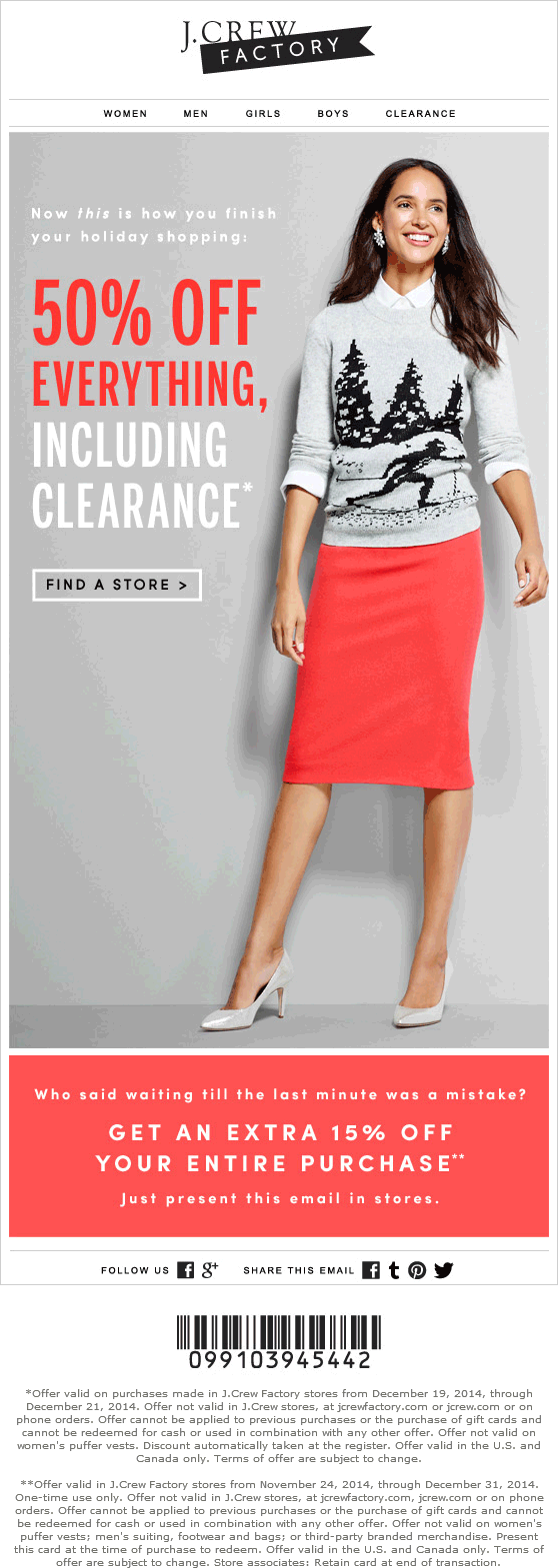This image is a detailed screenshot of the J.Crew Factory mobile website, characterized by a vertically elongated, rectangular layout. The top portion features a white header with "J.Crew" written in black capital letters. Adjacent to it, "Factory" is displayed in white text within a notched rectangle, resembling a ribbon. 

Below the header, a navigation menu with five items is present, although the small font renders them unreadable. Dominating the majority of the page is a large photograph, prominently showcasing a woman likely of Latino descent, inferred from her dark hair and skin tone. She is dressed in a very light gray sweater adorned with three black pine tree images and a small depiction of a skier, paired with a subtle red, almost pink, knee-length skirt. Her footwear consists of white flats with modest heels, approximately one to two inches in height.

On the left side of the image, bold red text announces a "50% off everything" sale, with "including clearance" in bold white font directly beneath it. Further down, "find a store" is displayed in black text. The overall background of the webpage is gray, transitioning to a pink border at the very bottom. Within this pink border, white text offers an additional "15% off your entire purchase," accompanied by unreadable fine print and a barcode directly above it.